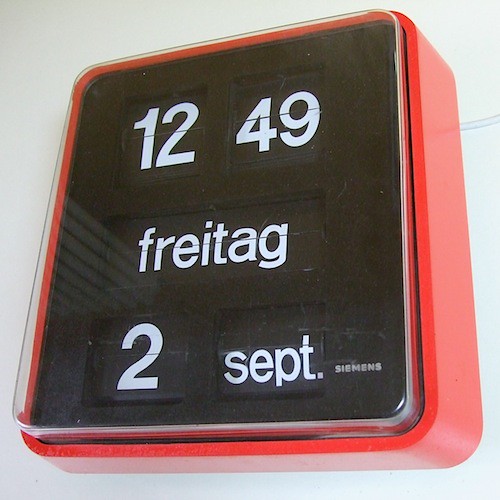This is a color photograph of a small, square wall clock with rounded corners, mounted on a white wall. The clock features a striking red plastic frame and a black face, covered by a plastic cover. The time displayed is 12:49, presented on white numbers against the black background. Below the time, the day is indicated in German as "Freitag" (Friday), and the date is given as "2 SEPT." The brand name "Siemens" is visible in the lower right-hand corner, confirming the manufacturer. The clock uses a mechanical display mechanism with flaps rather than an LCD display, adding a tactile element to its modern design.